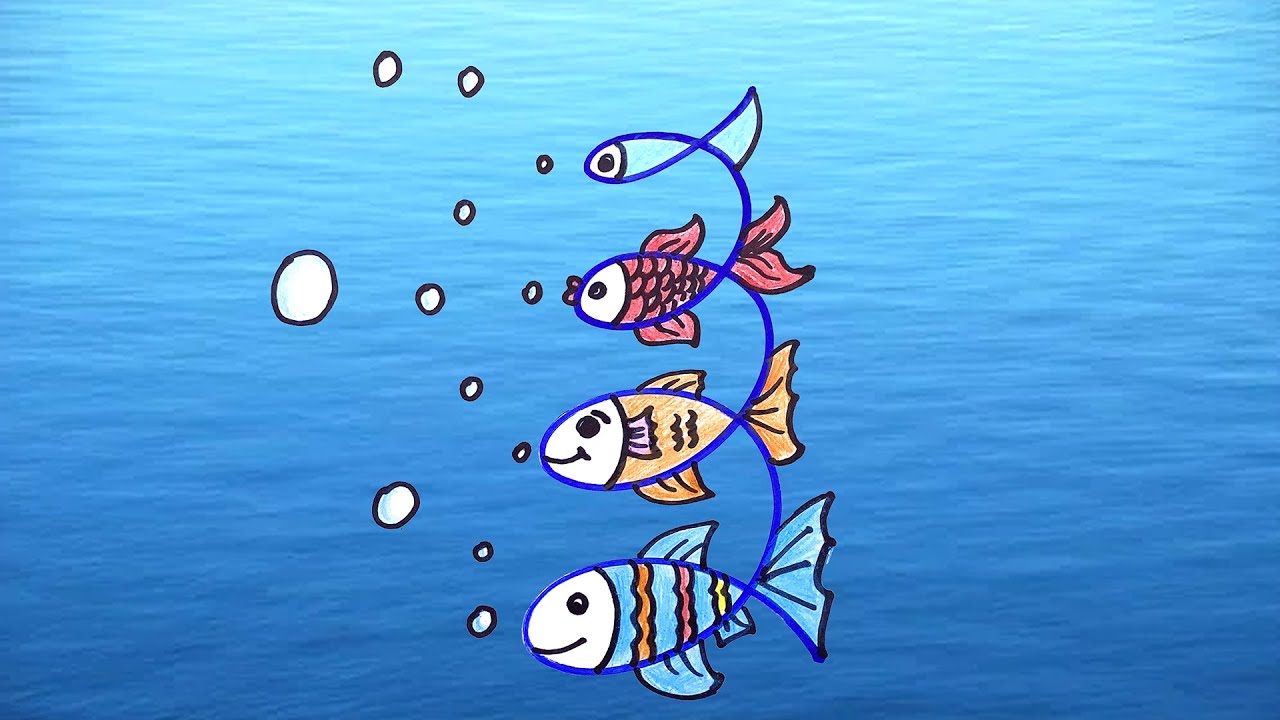This illustration features a whimsical, childlike depiction of fish within a vibrant aquatic setting. The background is a composite of a stock photo-style image of water, with gentle waves and light shimmering across its surface, shifting from lighter blue at the top to darker blue at the bottom. In the center, four cartoon fish are arranged vertically, each connected by a squiggly purple line that weaves amongst them. 

The fish are colorful and distinctly stylized, resembling drawings from a child's notebook. At the top is a slender, light blue fish with a single black eye. Below it, a slightly larger, red fish with red scales, a white face, a single black eye, and a small pink mouth. The next fish is orange with a white face, a smile, and distinctive pink fins. Finally, the largest fish at the bottom has a light blue body adorned with orange, pink, and yellow stripes, a white face, a cheerful black-lined smile, and a white eye. Cartoon bubbles, white and round, float upward in front of the fish, enhancing the playful, illustrative feel of the scene.